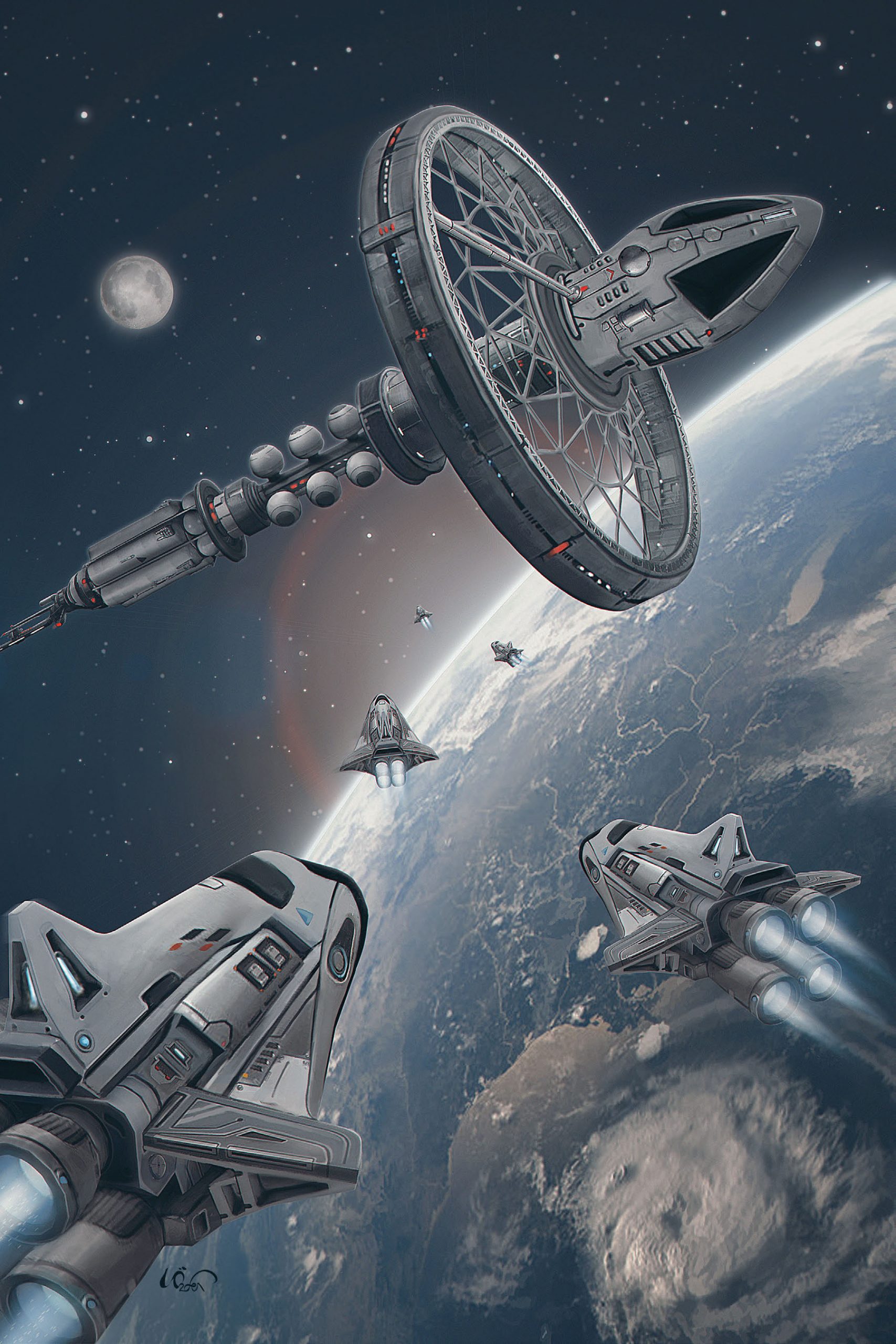This detailed illustration depicts a fleet of gray, fighter-pilot-style spacecraft orbiting above a planet that closely resembles Earth. Positioned predominantly on the right and center of the image, the planet showcases its vivid blue oceans, landmasses, and swirls of white clouds. The spacecraft are marked by their distinctive triangular shapes and four bright blue exhaust flames, trailing behind as they navigate through space.

In the foreground, three of these spacecraft appear prominently, their intricate designs highlighted, while two smaller ones are seen maneuvering further in the distance. Additionally, a large circular space station reminiscent of the "2001: A Space Odyssey" bike wheel design is visible, with a central post running through it, contributing to the scene's science fiction ambiance.

To the upper left of the composition, the moon hovers against the black, star-filled expanse of space, adding depth and contrast to the scene. The meticulous detailing and vibrant colors suggest this is a computer-generated painting, masterfully capturing the futuristic essence of interstellar exploration.